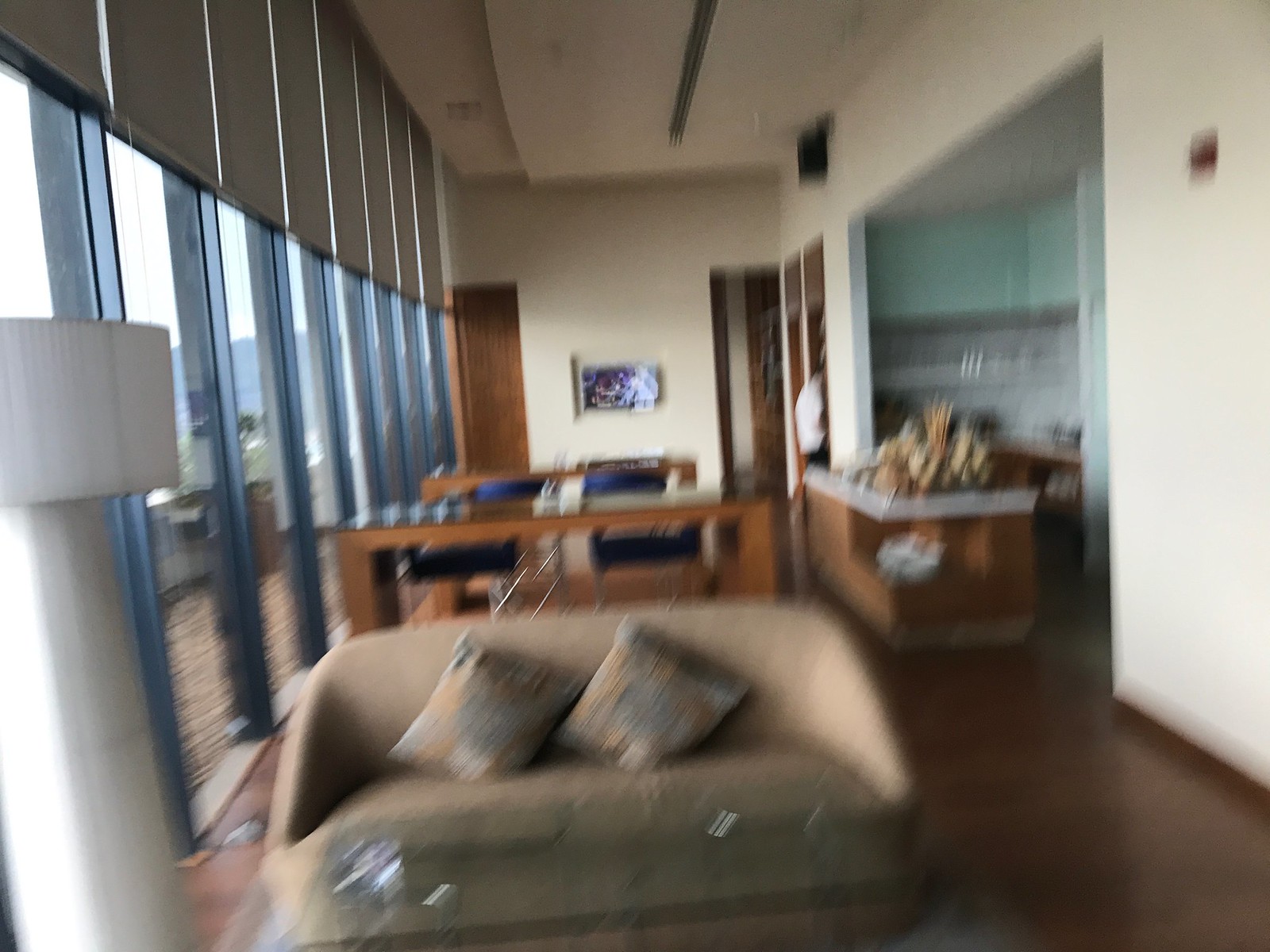This photograph captures a living room in mid-movement, resulting in a blurry and somewhat out-of-focus image. Dominating the left side of the scene are a series of large windows separated by blue beams, giving the room an open and airy feel. Instead of traditional curtains, roll-up cloth screens cover the windows. A white object, possibly a shelf, is also mounted on the windowed wall. 

The center-bottom of the photo features a rounded brown loveseat adorned with two pillows placed at an angle, creating a diamond-like arrangement. Behind the loveseat is a medium-colored wooden table or desk. The room's walls are painted in an off-white hue, providing a neutral backdrop. 

To the right, the living room opens up into what appears to be a kitchen. The kitchen walls are a combination of white and light mint-green colors. A bar-type countertop extends between the kitchen and the living room, serving as a visual and functional divider. On the far back wall of the living room, a painting or photograph is hung, adding a touch of artistic flair to the space.